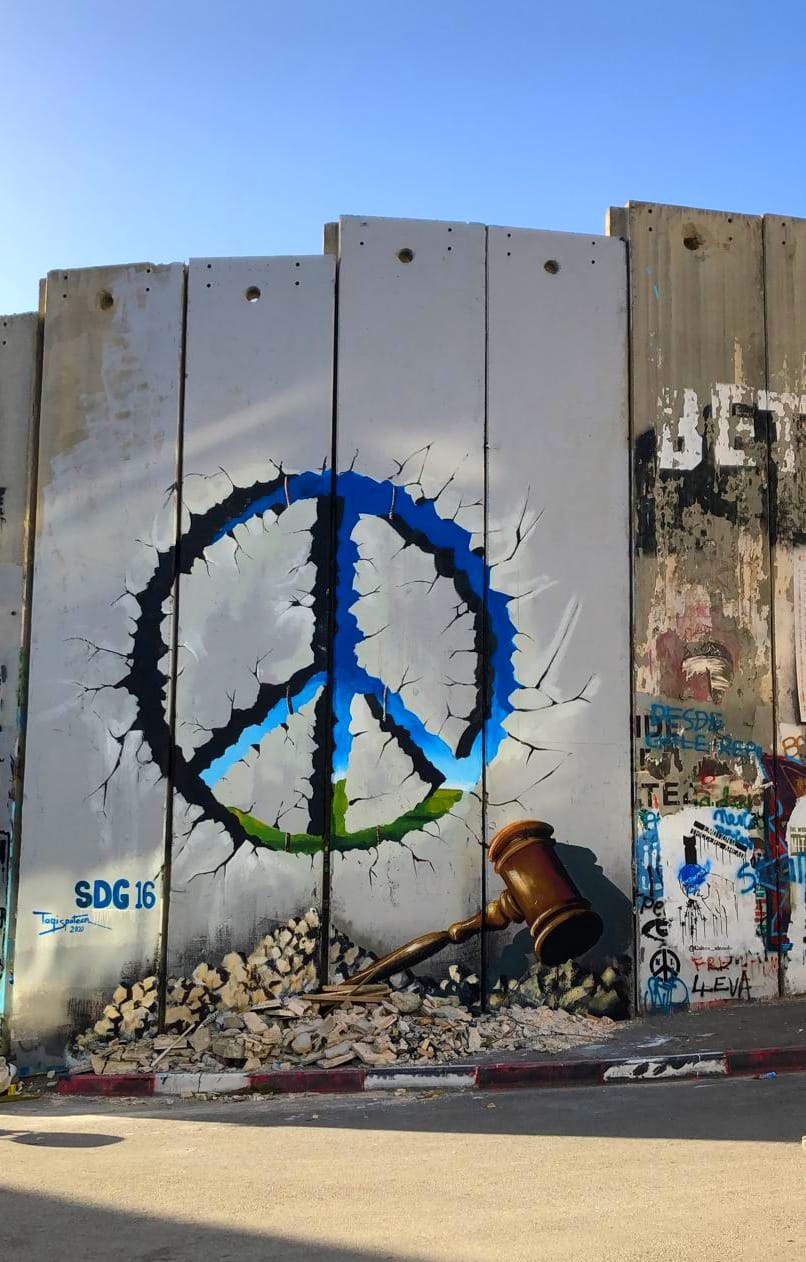The image showcases a detailed mural painted on the side of a wooden fence, some parts of which are painted white while others remain their natural wood color. The centerpiece of the mural is a large peace sign, painted with dark blue at the top, light blue in the center, and green at the bottom. The peace sign has noticeable cracks around it, adding a sense of wear and antiquity. Below the peace sign, near the bottom left, the text "SDG 16" is prominently displayed in blue, alongside a small signature. Scattered around the base of the fence are stones and a wooden mallet, reminiscent of a courtroom gavel. The mural is framed by various graffiti tags and letters in blue, black, and green, including another, smaller, black spray-painted peace sign. The background features a sunny sky with blue hues, adding light and contrast to the overall scene. The sidewalk and paved road in front of the fence are predominantly gray, with touches of red on the edge of the sidewalk, contributing to the urban aesthetic.